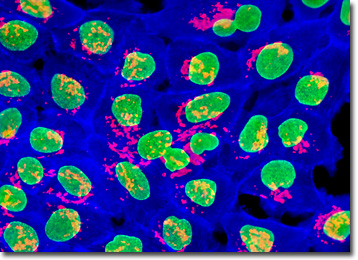The image captures an abstract portrayal reminiscent of plant cells or microorganisms under infrared light. Dominating the scene are numerous lime green blobs, each featuring bright yellow spots that appear almost luminescent, creating an otherworldly glow. These green structures are accompanied by scattered hot pink markings, as though paint has been splattered throughout, further enriching the visual complexity. Binding the elements together is a network of interwoven indigo blue splotches, blending seamlessly into a stark black background that adds depth to the image. The arrangement of colors—electric blue, lime green, hot pink, and black—is random and haphazard, suggesting a form of abstract art rather than a structured pattern.